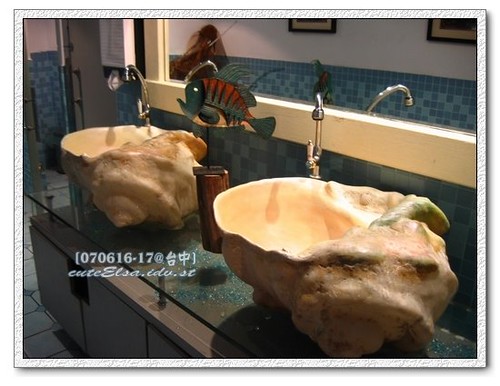The image depicts an elaborately decorated bathroom with a nautical theme. Central to the scene are two oversized conch shells used as sink bowls, into which arching silver faucets with single handles pour water, mimicking the flow into areas where snails would typically reside. The sinks rest on a green countertop trimmed in white, and below this countertop is a grey cabinet with multiple cupboards. A pivotal feature between the two sinks is a figurine of a green fish with red and black stripes, possibly metallic. Above the sinks, a cream-framed mirror occupies much of the right wall, reflecting glimpses of two pictures and a dispenser to its left. Wainscoting with wallpaper runs along the lower part of the walls, complemented by aqua ceramic tiles in varying shades of blue, creating a cohesive, seaside atmosphere. The bottom edge of the mirror reveals a cryptic text—"070616-17 Cute Estal IDU Southeast"—which seems like an advertisement for the unique seashell sinks.